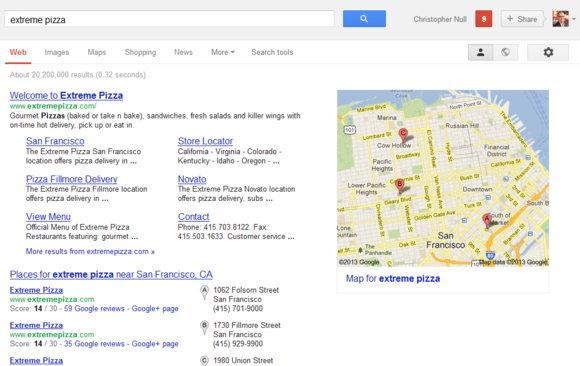The web page displays a search query for "Extreme Pizza" entered into a gray search bar positioned at the top of the page. The search bar features a blue button labeled "Search." Below the search bar, the word "web" is highlighted in red, accompanied by a welcome message that reads, "Welcome to Extreme Pizza." 

The page provides various locations, the first of which is San Francisco. The details for this location include options such as "Pizza Fillmore Delivery," "View Menu," and "Store Locator." There is also information about a Nevada location with a note that it offers pizza delivery, accompanied by a "Contact" section and a phone number for Extreme Pizza.

Beneath this, there’s a section titled "Places for Extreme Pizza near San Francisco," listing three nearby locations. 

To the right of this information, presented on a white background, is a sizeable square map displaying the San Francisco area. The map features several red pins marking the Extreme Pizza store locations. Below the map, a blue caption reads, "Map for Extreme Pizza."